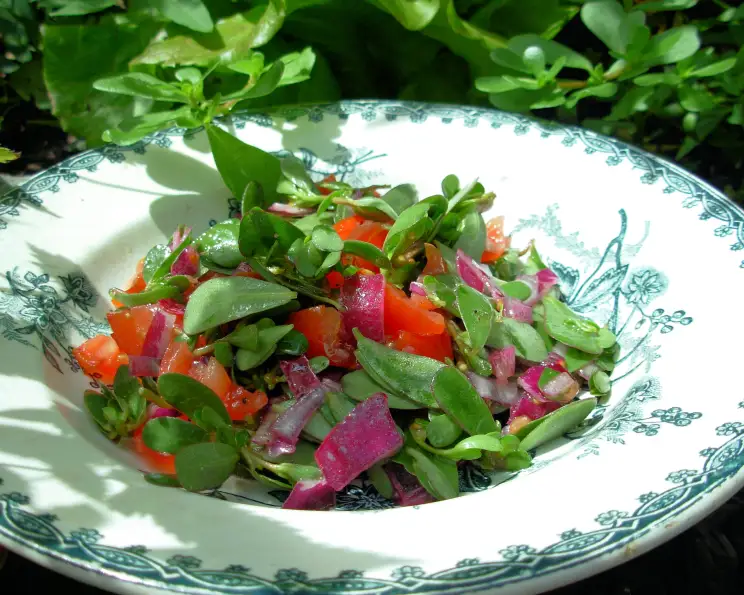This image captures a vibrant summer salad artfully presented in a white ceramic plate with intricate emerald green floral and foliage patterns, reminiscent of Delphware. The salad, bursting with color, features an assortment of young greens, sliced tomatoes, red onions, and possibly radishes and snap peas. The plate is set against a lush background of greenery, suggesting it is placed outdoors, basking in sunlight, which enhances the fresh and healthy appeal of the dish.